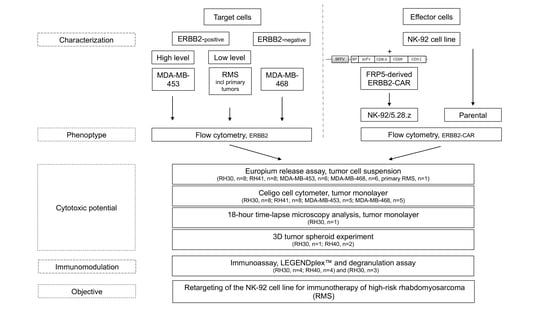This detailed black and white flowchart visually organizes the characteristics and interactions of target cells and effector cells, accentuating their roles in cancer research. On the left side, the chart lists several key attributes of target cells, including characterization, phenotype, cytotoxic potential, immunomodulation, and objectives. On the right side, a parallel section details the distinct traits of effector cells, notably featuring the NK92 cell line, which directs towards parental flow cytometry. The two sections converge, depicting shared characteristics through arrows pointing towards a series of tables and processes such as flow cytometry, europium release assay, tumor cell suspension, and 3D tumor spheroid experiments. With boxes meticulously outlining each element, this diagram succinctly illustrates the methodical breakdown and comparison of specific cell properties crucial for understanding cancer behaviors and therapies.